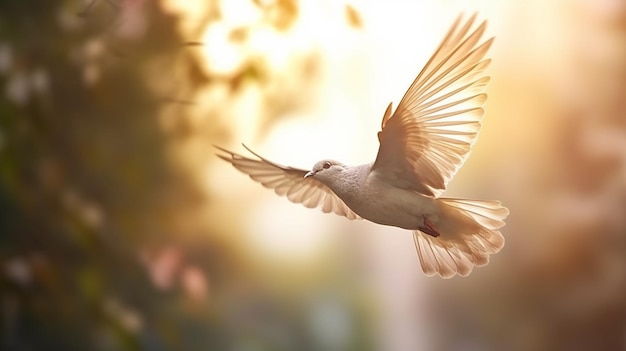In this vibrant outdoor photograph, a white dove is captured in mid-flight, positioned slightly right of center as it glides towards the left. The dove's wings are fully extended, showcasing the intricate details of each feather, while its tail feathers are fanned out behind, adding to the elegance of its form. The bird’s body and head are entirely white, adorned with subtle tan accents on its feathers and underbelly. Its dark eyes and pointy beak are clearly visible. The dove’s feet are tucked in and extended towards its back. The background is artistically blurred, enhancing the focus on the dove. However, hints of the background reveal a bright white sky, possibly illuminated by the sun, with blurred trees and shrubs on either side. The trees on the left side appear to have pink blossoms, adding a splash of color to the serene scene. Overall, the photograph beautifully captures the dove's grace and purity in mid-flight.